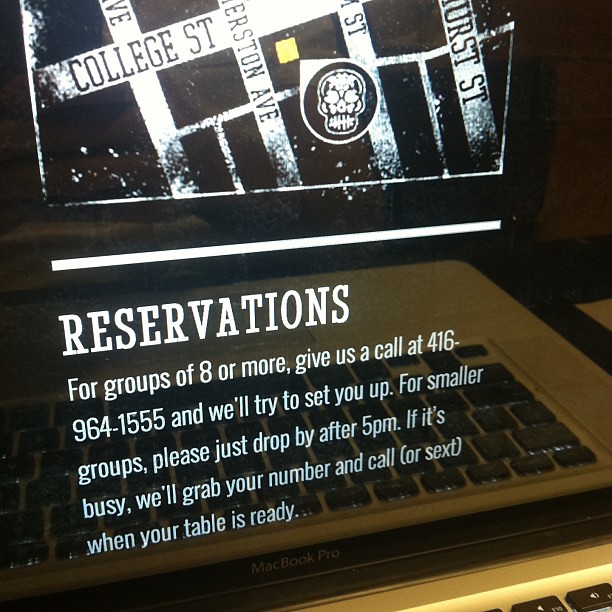The image is a promotional photograph for a restaurant, displayed with white text on what appears to be a glass surface in front of a computer keyboard. The top third of the image features a partially visible map with the words "College Street" prominently shown, alongside other street names that are cut off, making them unreadable. A skull emblem is also visible on the map, likely indicating the restaurant's location. The white text overlaying the keyboard reads: "Reservations" in bold, followed by a detailed announcement. It states, "For groups of eight or more, give us a call at 416-964-1555 and we'll try to set you up. For smaller groups, please just drop by after 5 p.m. If it's busy, we'll grab your number and call (or sext) you when your table is ready." The text and map together create a detailed and intriguing advertisement for the restaurant.